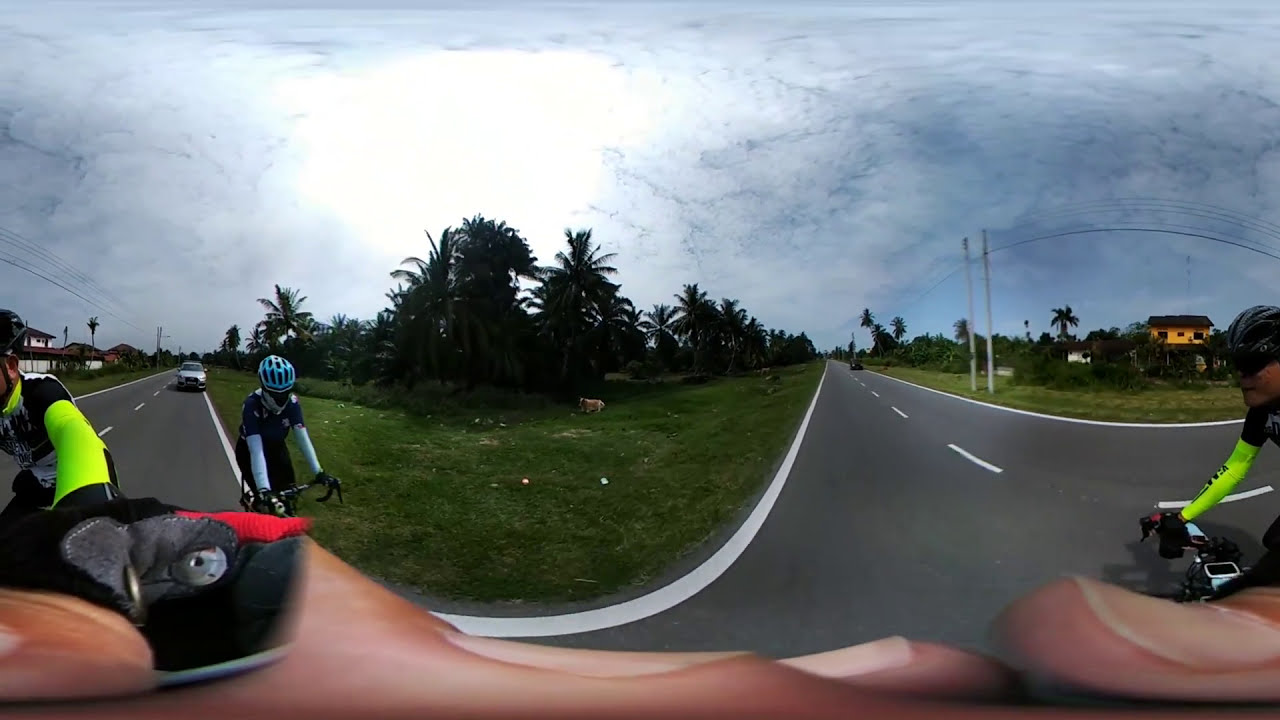This detailed 360-degree photograph, likely taken by a pedal biker with a camera mounted on the handlebars, captures a dynamic scene of cyclists on a winding road that appears distorted into a U-shape. Central to the image, we see two cyclists—one wearing a black cycling uniform with neon yellow sleeves and a black helmet, and another in a navy blue shirt with long white sleeves and a light blue helmet. Their positions in the warped image suggest they are the same individuals seen from different angles. Directly below, the photographer's close-up fingers slightly obscure the view, emphasizing the handheld nature of the shot. A silver car is visible in the background, trailing the cyclists on the black-topped road marked by solid white lines along the edges and dashed white lines in the center. Lush, green grass flanks both sides of the road, complemented by tall palm trees that evoke a Southern locale, possibly Florida. A house with yellow siding and brown roofing is situated to the right, while white structures and a white house with brown shingles can be seen to the left. The blue sky above, tinged with ominous clouds, hints at impending rain, adding a layer of atmosphere to the vivid roadside scene.